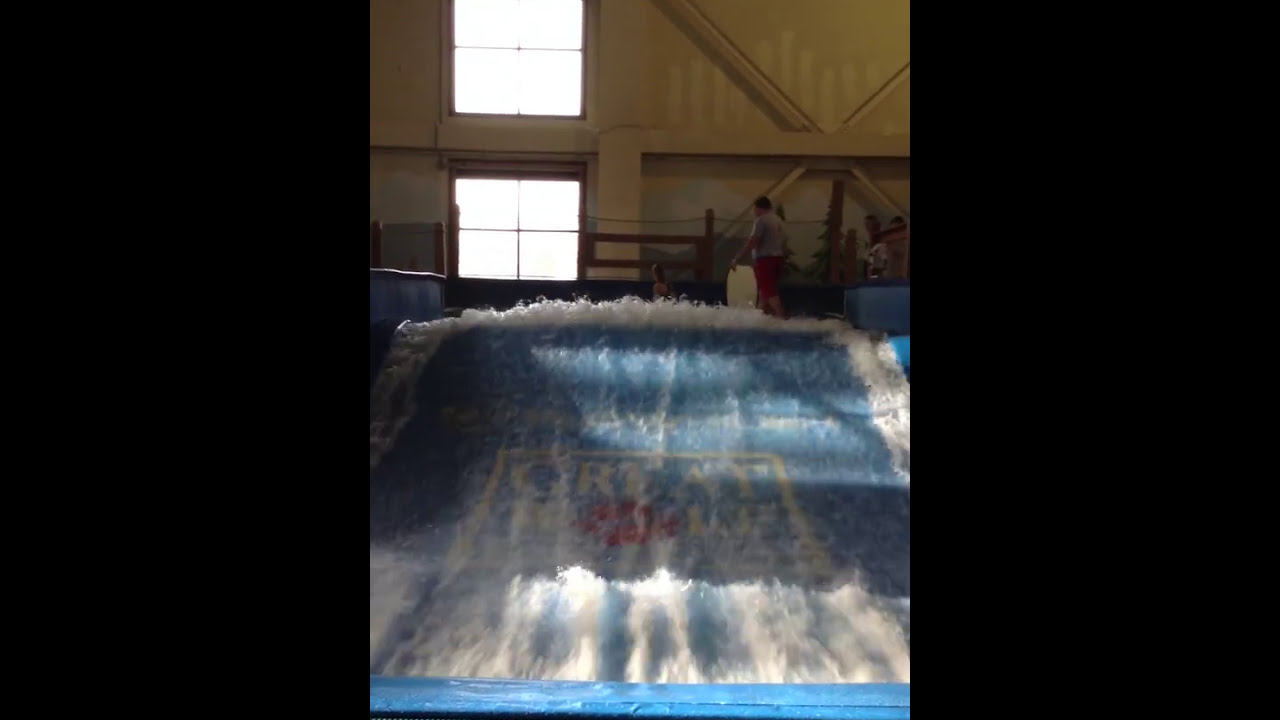The image depicts an indoor water park scene, centering on a blue-colored boogie board simulator. The simulator features water rushing at an angle, creating foamy waves. In the foreground, a man dressed in red shorts and a grey shirt, holding a yellow boogie board, is about to take his turn. A blue lining outlines the wave simulator, and the water's surface partially obscures a logo, making it difficult to discern specific letters. The background reveals a white wall with two glary windows aligned vertically and sunlight streaming in, creating a bright atmosphere. Additional people can be seen milling about, some likely waiting for their turn on the simulator. The overall scene captures the energetic and vibrant environment of the indoor water park.